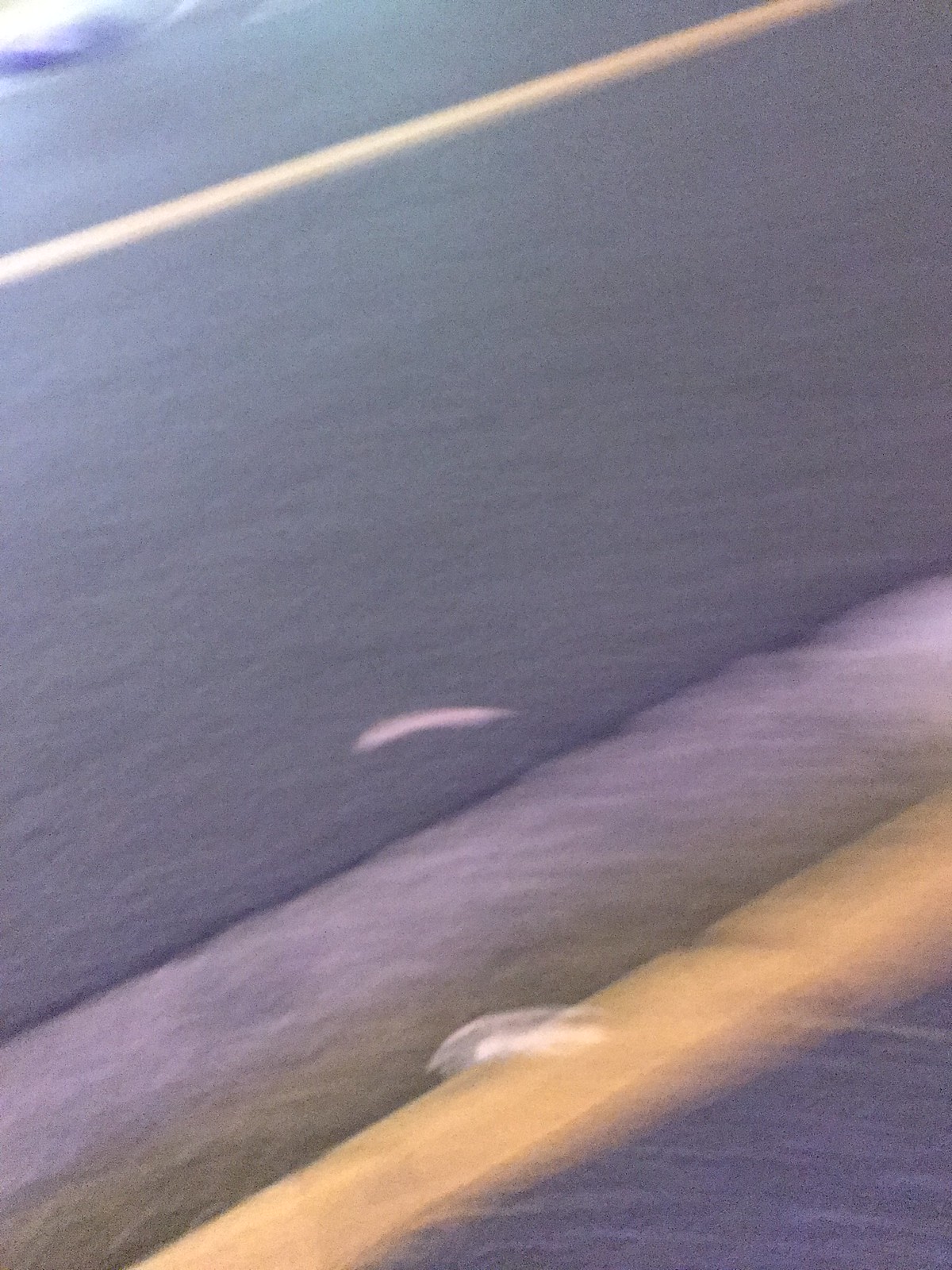This blurry, color photograph captures a nighttime street scene from a first-person point of view, possibly taken from inside a car or by someone walking on the pavement. The camera angle is slightly tilted downward, with the lens facing the road. The image is dominated by dark gray asphalt roads with a distinct yellow solid line running through the center, separating two lanes. On the bottom right of the image, there is a dark gray concrete sidewalk and a yellow diagonal curb that extends towards the center. Nearby, a small patch of grass can be seen on the road next to the yellow curb. The upper left corner of the image is illuminated, possibly by a street lamp or store light, adding a bright spot amidst the otherwise dimly lit scene.